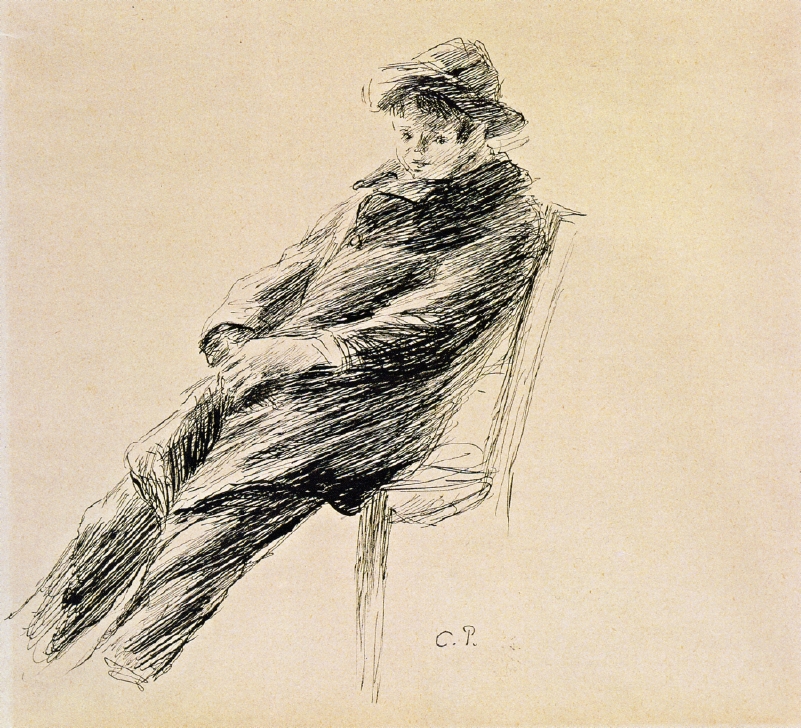This is a detailed, black and white drawing on beige paper, depicting a young boy sitting diagonal across a white chair. His body is relaxed, with legs stretched out straight in front of him and hands folded below his stomach. The boy is dressed in dark clothing, including a hat with a brim reminiscent of a raincoat, a dark coat, and dark pants. The chair's design is simplified, almost sketched loosely, which makes it appear partly undefined. The boy has a slightly wistful expression, with his bangs peeking out from under his hat as he gazes downward, perhaps at the artist. The artwork, signed "C.P.," appears aged, adding to its striking and evocative nature.